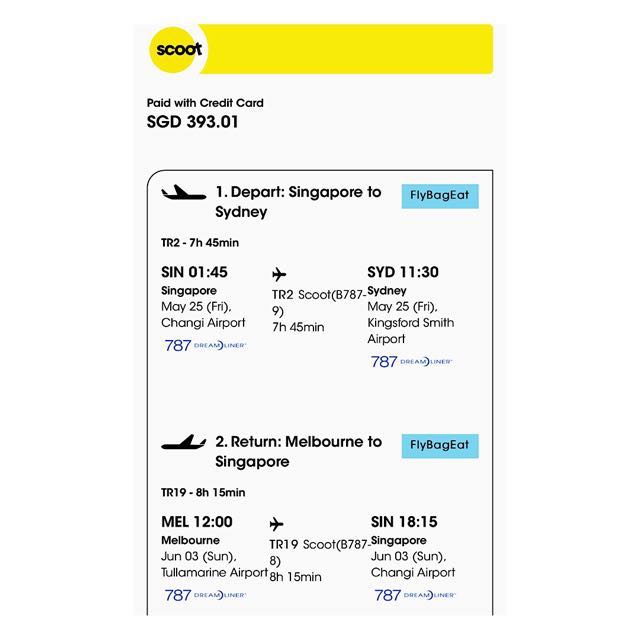In this image, set against a pristine white background, we see a detailed screenshot with prominent elements. At the top, a yellow circle with the word "SCOOT" in bold, black text serves as the header. Below this, in bold black text, is the statement "PAID WITH CREDIT CARD SGD 39301" set against the same white background. 

Directly below, outlined with a thin black border, is a box containing an icon of an airplane in black, pointing east. Adjacent to the icon is the label "Number 1, DEPART, Singapore to Sydney." Additionally, there is a prominent blue action button on the right side, labelled "FLY BAG EAT." Following this, text indicates flight details with "SIN 145" and "SID 1130" positioned side by side.

Further down, the return flight details are presented, with another airplane icon facing west, indicating the direction of the return journey.